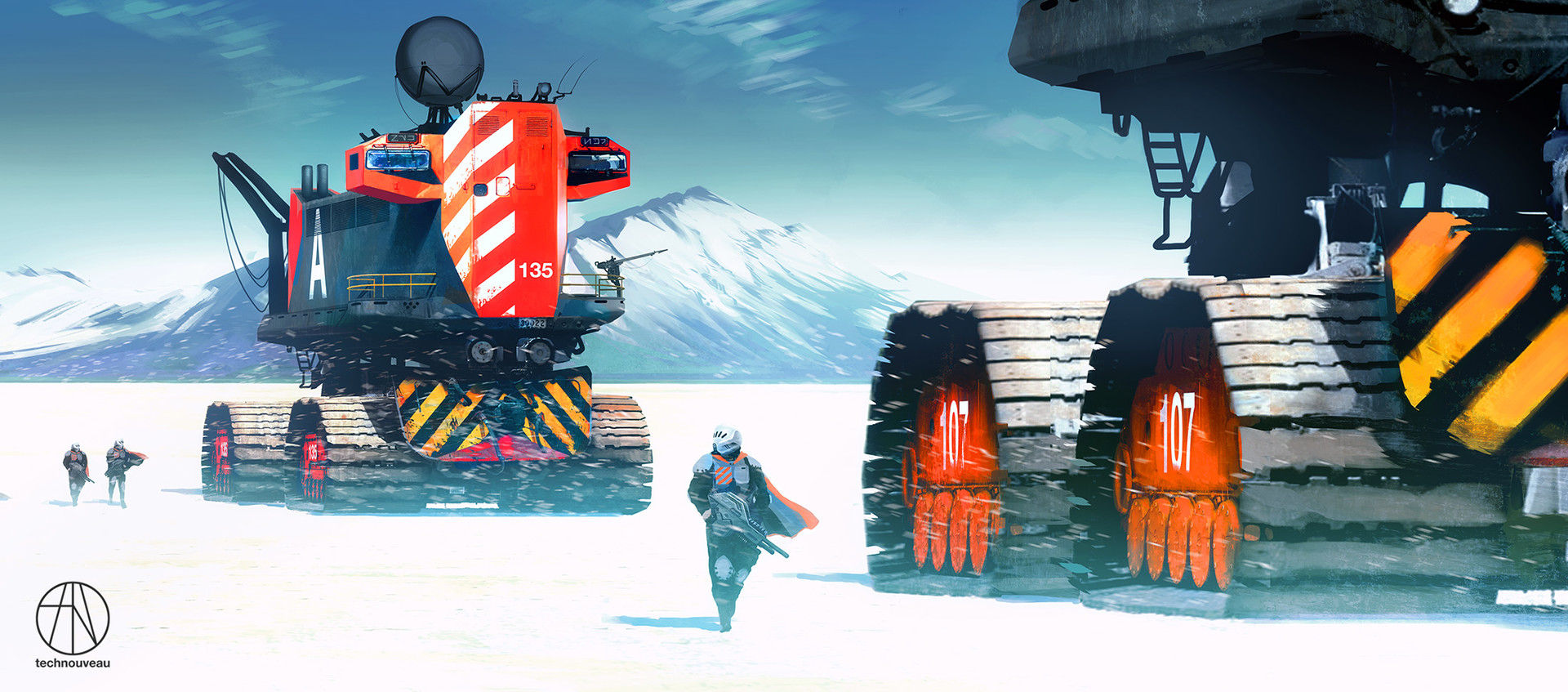This digital artwork depicts a futuristic sci-fi scene set in a cold, Arctic-like tundra with a clear, snow-covered expanse stretching towards the horizon. Dominating the background is a majestic, blue and white snow-capped mountain under a clear blue sky. Scattered throughout the image are two colossal, tank-like machines with sturdy gray treads and distinctive orange studs. The vehicle closest to the viewer, partially cropped on the right side of the frame, has a gray body with striking orange and white designs, marked prominently with the number '135' in white on the front and a large white 'A' on the side. This vehicle also features a yellow and black hazard stripe, adding to its industrial look. In the center of the scene, standing atop the snowy ground, is a figure clad in futuristic gray armor and a matching helmet, adorned with an orange and gray cape. Flanking this central figure, two additional people dressed in similar garments stand to the left, each appearing to carry weapons and wear capes, contributing to the militaristic feel of the scene. The image's detailed rendering showcases a stark, wind-swept environment, with the high-tech machines and heavily-armored individuals suggesting a blend of advanced technology and extreme climatic conditions.